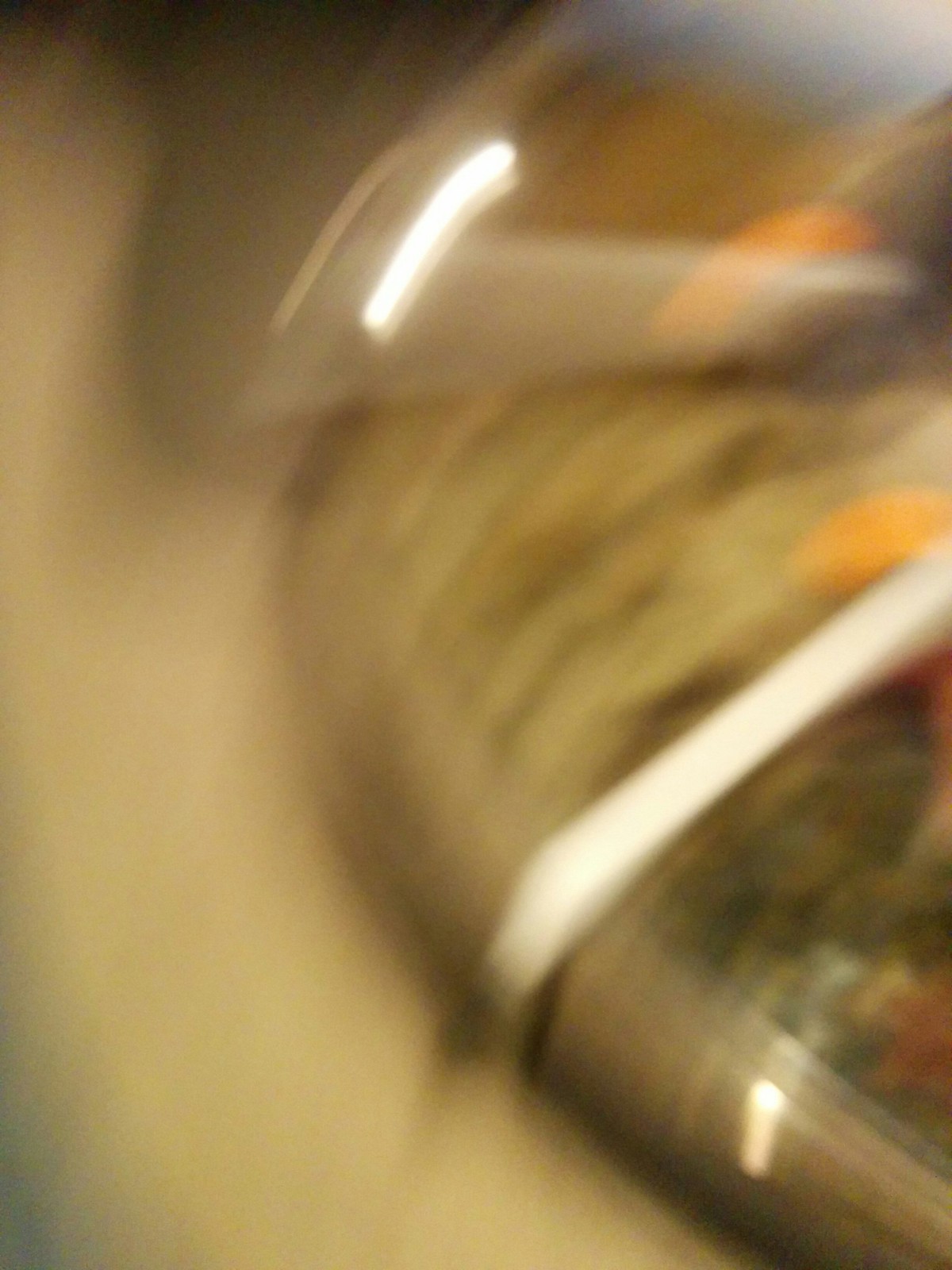The photograph is a highly blurry, vertical rectangular image, seemingly capturing a section of a salad bar at a buffet. The blurriness suggests the camera was moved in a diagonal motion from the lower left to upper right. The image shows a container with lettuce, with its green hues and orange smudges possibly indicating other salad ingredients like orange wedges. The top right side of the photograph features a rounded object, enclosed by a dark gray border, intersected by two light gray straps. Despite the image's overall mustardy and light beige tones, suggestive of the surface or the ambiance, the salad bar elements stand out. The scene is further characterized by reflective qualities, hinting at glass or plastic surfaces within the salad bar's setup.